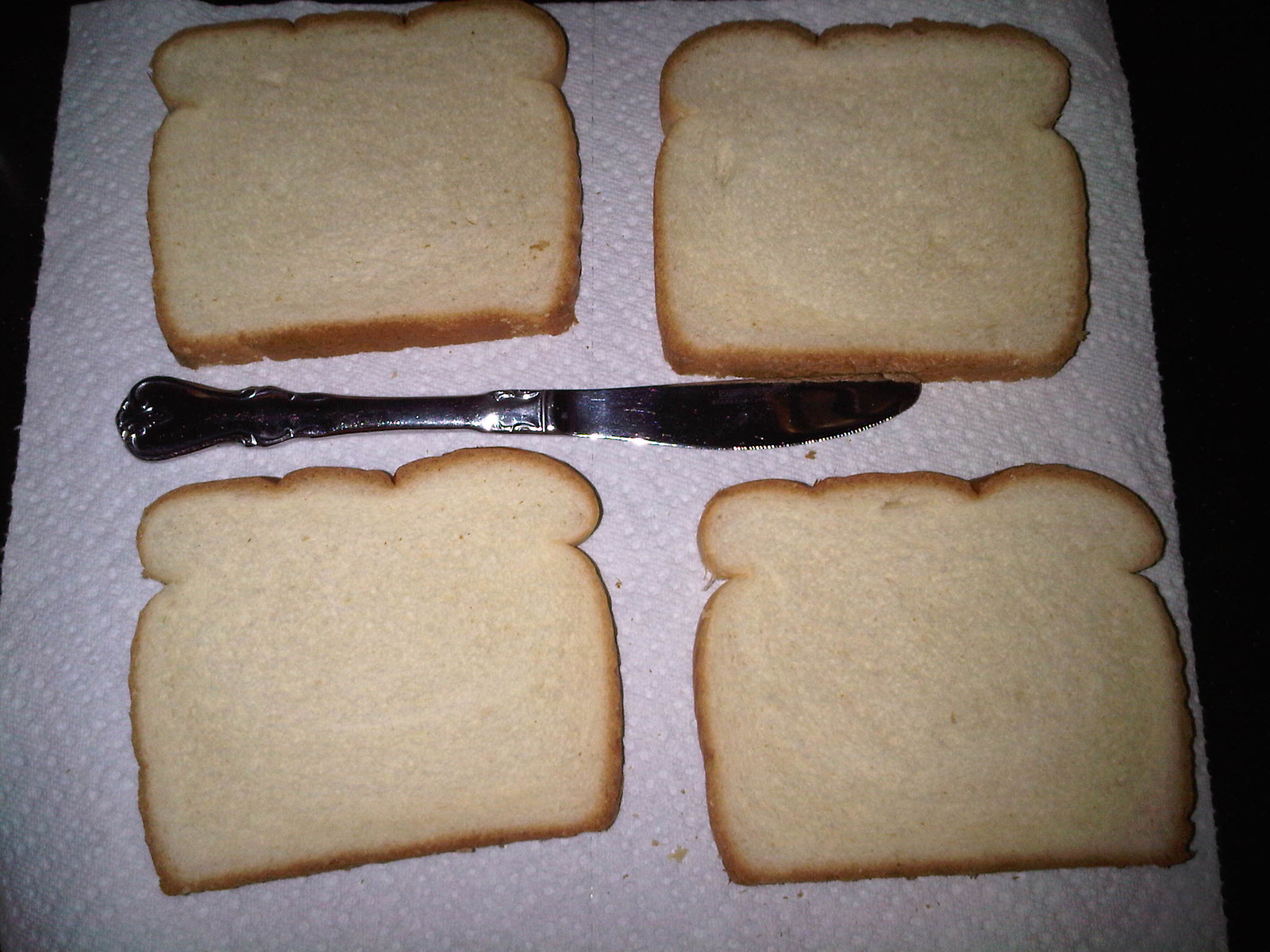This detailed photograph captures four pieces of typical white sandwich bread with brown crusts, neatly arranged in a square formation on a plain, white paper towel with visible dotted texture. The bread is unbuttered and untoasted, with crumbs scattered around on the paper towel. A decorative silver butter knife is placed horizontally between the top and bottom pairs of bread slices, with its blade pointing to the right. The background of the image is predominantly black, visible as thin slivers on the left and right sides, accentuating the simplicity of the scene.